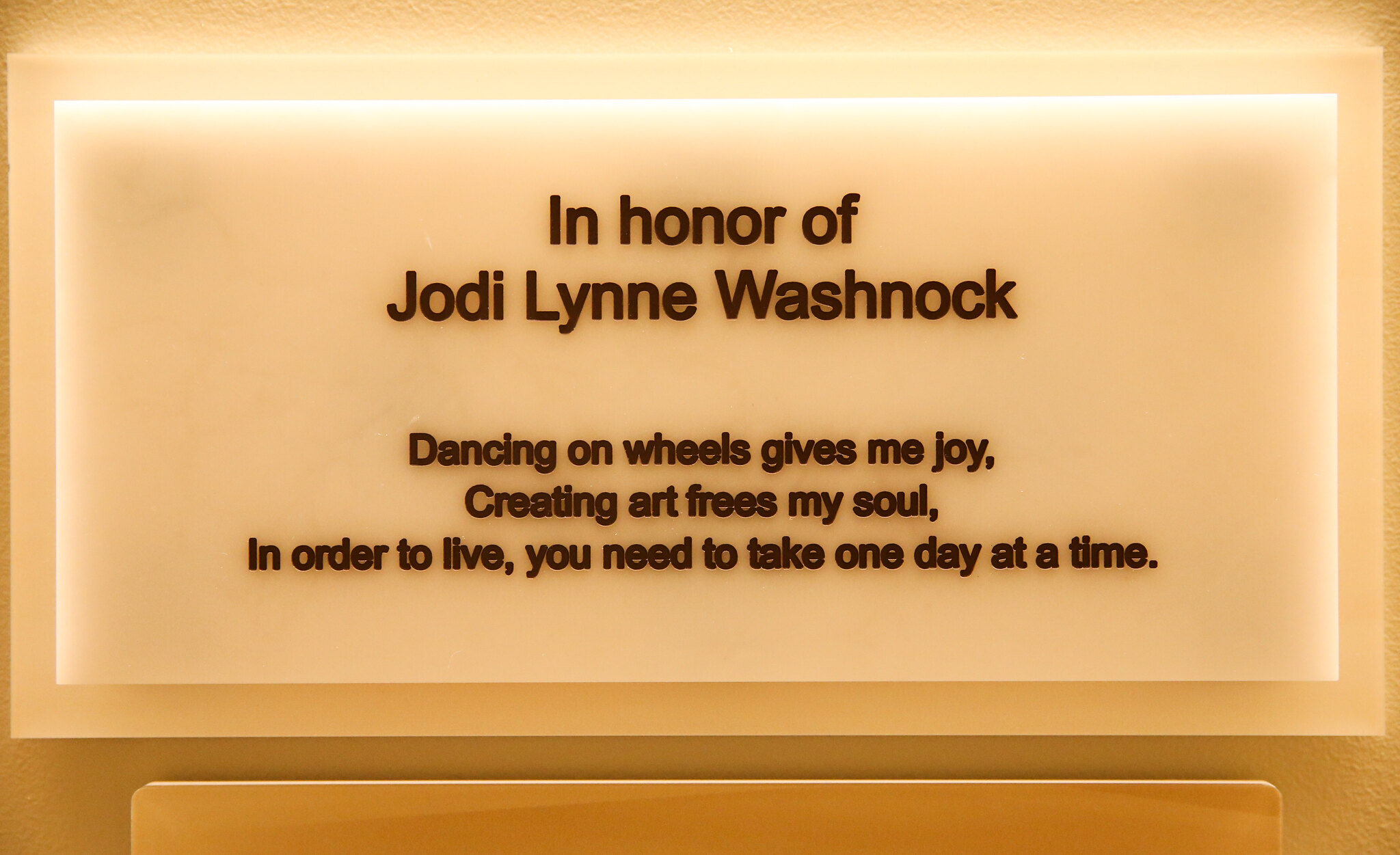The image features a close-up of a memorial plaque, mounted on a light brown, stone-like background. The plaque itself is constructed from semi-translucent white marble or alabaster, and it is illuminated either from above or possibly backlit, adding a subtle glow to its surface. The inscription on the plaque is in black text and reads: "In honor of Jody Lynn Washnock." Below this, in smaller black text, it continues with the heartfelt words: "Dancing on wheels gives me joy, creating art frees my soul. In order to live you need to take one day at a time." The plaque is set within a thin border, possibly darker in color, which contrasts with the light stone surface that forms the broad background. Despite varying opinions on its visual appeal, the plaque aims to capture the essence and spirit of Jody Lynn Washnock’s life and passions.